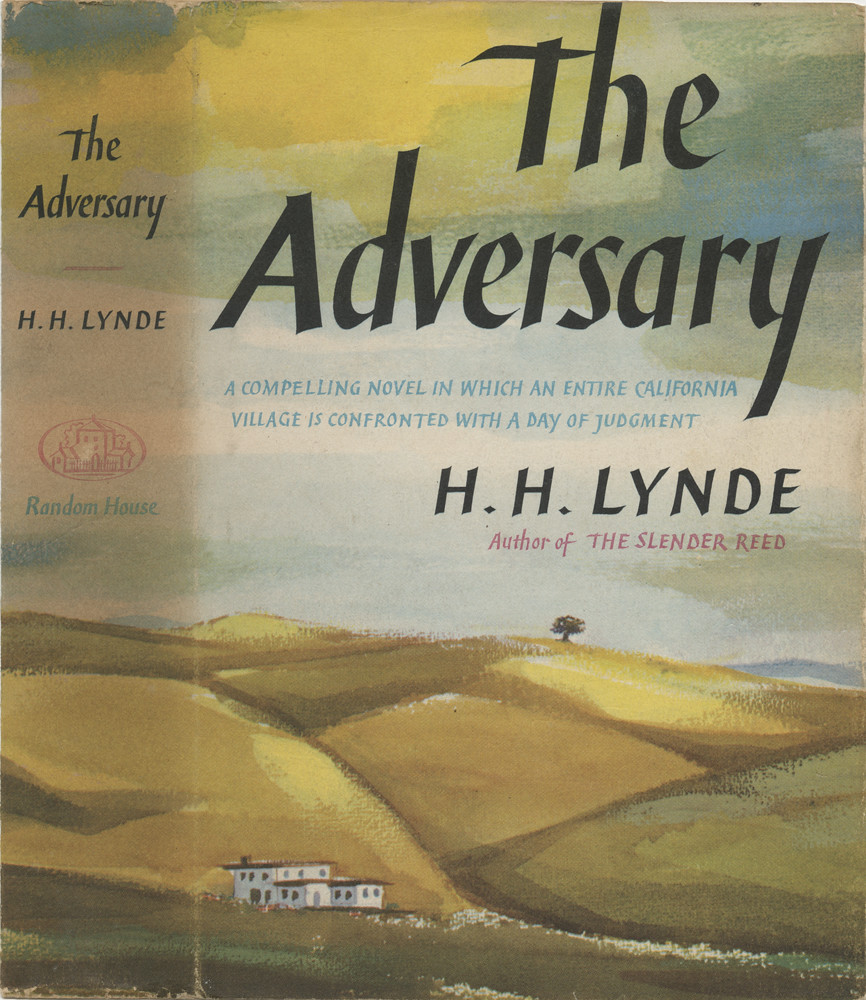The image depicts the front cover of an older hardback book titled "The Adversary" by H. H. Lind, published by Random House. The book cover features a painted countryside scene with golden-yellow hills and a single white, two-story house with a brown roof situated on the hillside, accompanied by two smaller one-story houses with windows. A solitary tree stands majestically on the top of the highest hill, adding to the isolated and contemplative atmosphere. The sky above is a mix of grays and greens, with touches of yellow at the top, setting a somber tone. In bold black letters at the top left, the title "The Adversary" and the author's name "H. H. Lind" are prominently displayed. Beneath the title, in smaller blue print, appears the tagline: "A compelling novel in which an entire California village is confronted with a day of judgment." The author's name, H. H. Lind, is repeated in larger bold black print, followed by a note in red indicating Lind as the author of "The Slender Reed." The spine of the book also displays the title and author's name, "The Adversary, L. L. Lind," ensuring visibility when shelved.